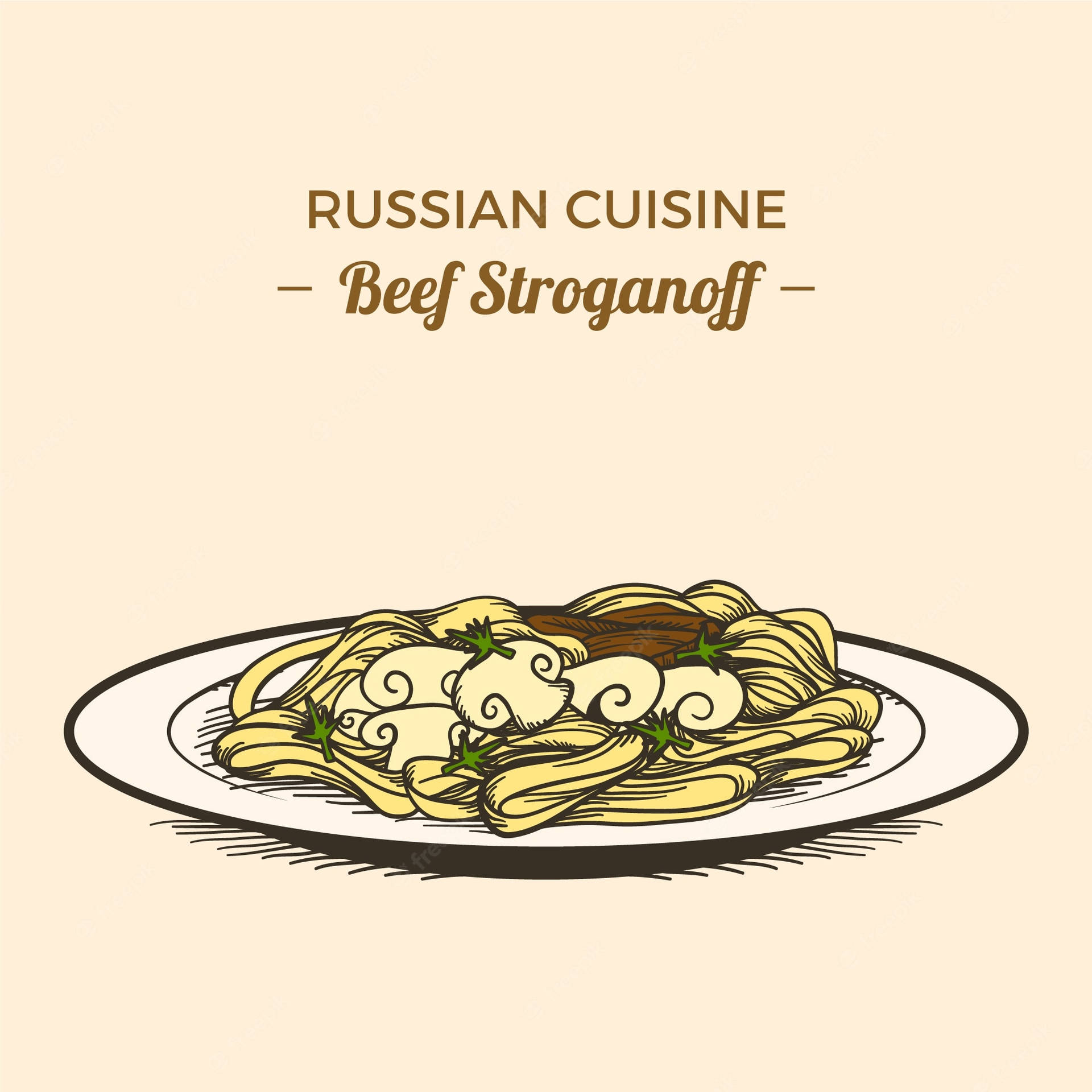The image is a stylized drawing with a simplistic look. The background is beige in color. At the top center, in warm brown and orange tones, the text reads "Russian Cuisine." Below this, in cursive, it says "Beef Stroganoff," flanked by dashed lines. The main focus of the image is a white plate featuring a black border and a subtle shadow underneath, giving it a slightly three-dimensional effect. On the plate, there is a serving of yellow pasta topped with beige mushrooms, garnished with green herbs that look like parsley or cilantro. Near the right side of the plate, there are flat brown meatballs arranged neatly. The overall color palette of the image comprises warm, neutral tones, enhancing its appealing aesthetic.